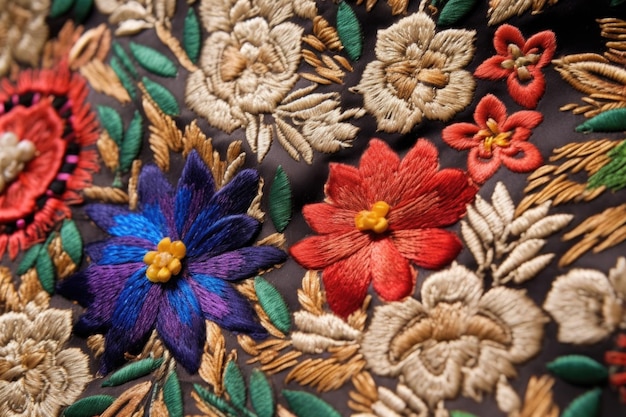This photograph showcases an intricate and elaborately embroidered piece of fabric, potentially velvet or macrame, with a dark brown or black background that features slight waves in the material. The embroidery presents a rich cornucopia of flowers and plants, executed in coarse threads that add texture and depth. The central focus includes several vividly colored flowers. Notably, there is a deep royal blue and purple flower with yellow pistils composed of small thread balls. To its right, a striking red flower with shades of deep and muted reds and oranges also has a yellow center. Surrounding these centerpiece blooms are additional flowers in beige, orange, and gold, alongside varied green and gold leaves. Tiny red flowers are scattered near the top, adding to the complexity and beauty of the composition. The balance of colors and the careful, detailed embroidery create a visually stunning piece of art.